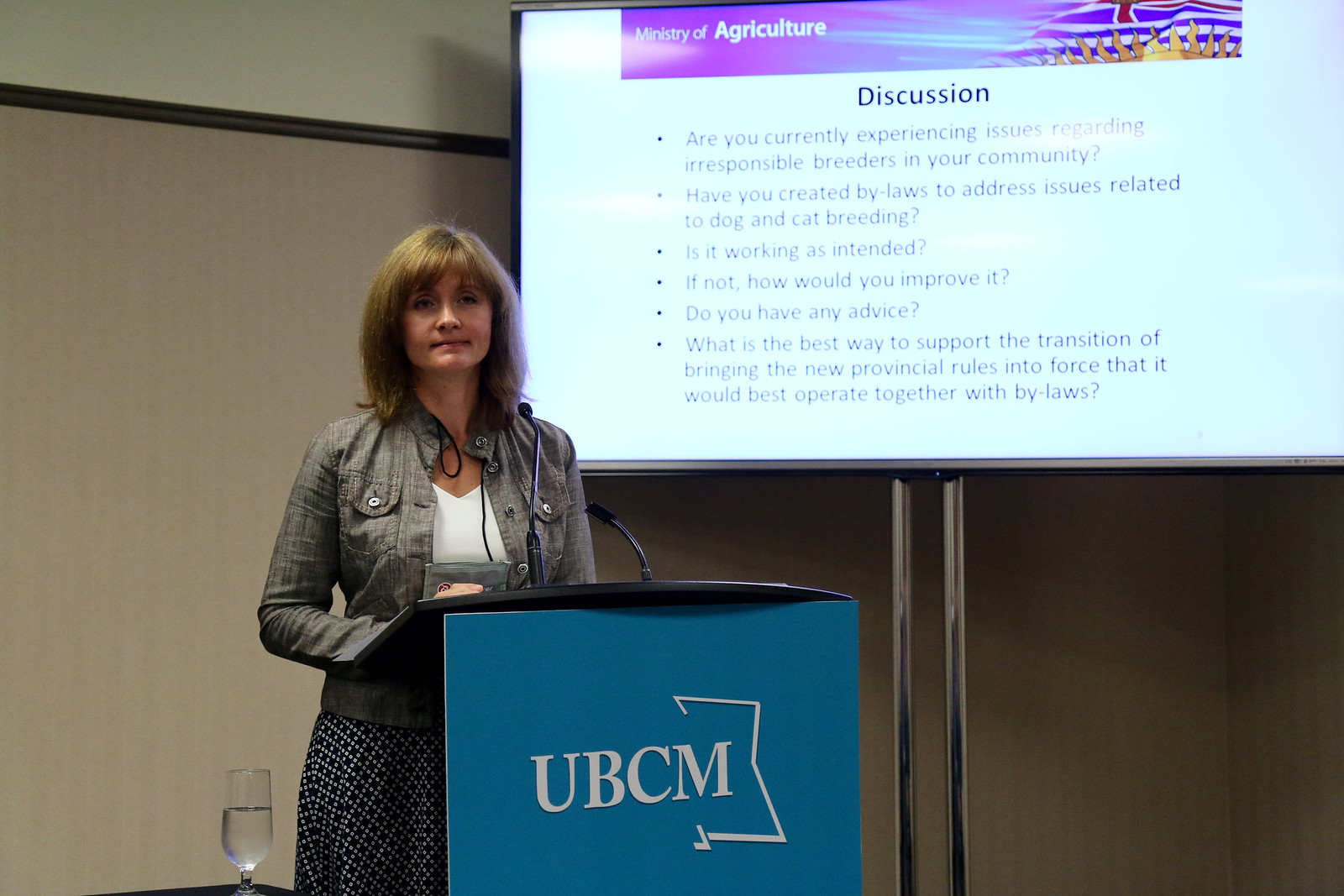A woman in her 40s with dirty blonde, medium-length hair featuring bangs, stands behind a blue podium labeled with white characters 'UBCM' and an accompanying illustration. She's dressed in a gray denim jacket, a white top, and a blue polka dot skirt. To her left, a glass of water sits on the podium. She appears to be giving a presentation, indicated by her stance and the presence of microphones. Behind her, a large silver-edged television screen displays a slide on a white background. The screen's text includes the heading "Ministry of Agriculture" and outlines several discussion points in black text: "Are you currently experiencing issues regarding irresponsible breeders in your community? Have you created bylaws to address these issues related to dog and cat breeding? Is it working as intended? If not, how would you improve it? Do you have any advice? What is the best way to support the transition of bringing the new provincial rules into force that it would best operate together with bylaws?"